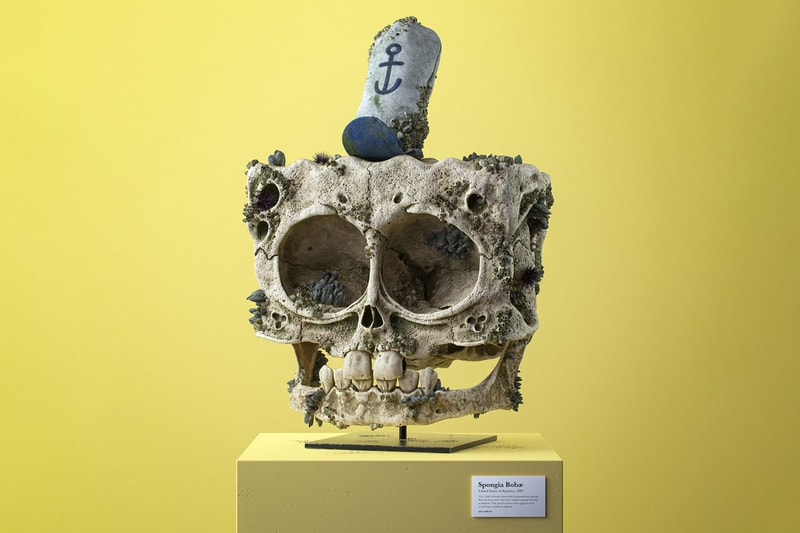This image depicts an intriguing sculpture that appears to be an artistic interpretation of SpongeBob SquarePants. The sculpture, situated on a yellow pedestal with a white plaque reading "Spongy a Babe," resembles a fossilized or stone skull. It has a distinctly square-shaped head akin to SpongeBob's, featuring deep inset eye sockets with rocks inside, a pair of large upper teeth, and four smaller lower teeth within an open jaw. The head is notably massive and squared, with hollow cheeks and a small nose, and is covered with moss-like or weedy green substance. Atop the skull rests a small white hat with a blue brim and an anchor emblem. The sculpture is on display in a museum setting, mounted on a black stand, against a yellow background that matches the base.